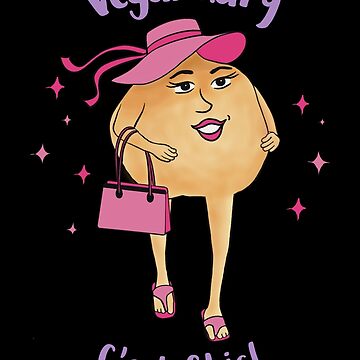This digital or marker drawing features a whimsical, ball-shaped character, reminiscent of an onion in shape. The character is depicted in a round, tan-colored form with exaggerated facial features—large eyes, pink lips, a white mouth, and eyelashes—all occupying most of its body. The figure is facing slightly to the right and downward. 

Adorning the character is a pink hat with a ribbon cascading off it, and it sports a pair of pink sandals. Hanging over its right arm is a rectangular pink purse with a black latch, adding a touch of accessorizing to its appearance. Surrounding the character are pink and light pink stars, creating a playful and dreamy atmosphere.

The background is entirely black, making the character and its accessories pop. At the top and bottom of the image, there are pink words, but they are partially cut off by the photo. This simplistic yet charming illustration captures the essence of lighthearted fashion and character design.